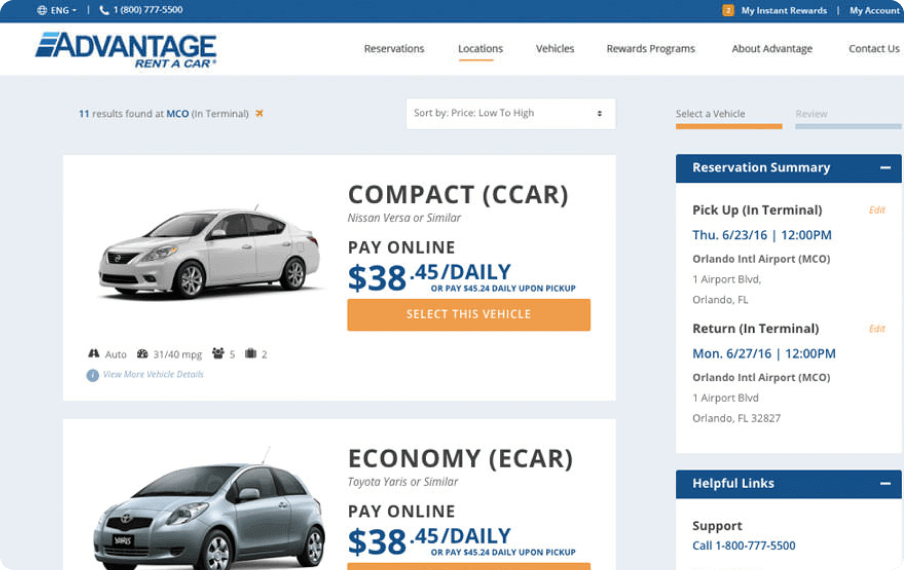This is a webpage for Advantage Rent-A-Car. The top of the page features a blue border with the text "English" and the customer service number "1-800-777-5500." Adjacent to this, there are links for "My Instant Reward" and "My Account." 

On the left side under the blue border, there is a menu with the following options: "Reservation," "Location," "Vehicles," "Reward Program," "About Advantage," and "Contact Us." 

Beneath the menu, in a light blue section, the text "11 results found at MCO and Terminal" is displayed. A sorting option follows, allowing the user to "Sort by Price, Low to High."

Below this section, there are two vehicle options presented with accompanying images:

1. The first vehicle is labeled as "Compact, C-Car, Nissan, Versa or similar." The pricing details show two options: "Pay online $38.45 daily" or "Pay $45.24 daily upon pickup." An orange button below this vehicle states "Selected Vehicle."

2. The second vehicle is labeled as "Economy, E-Car, Toyota, Yaris or similar."